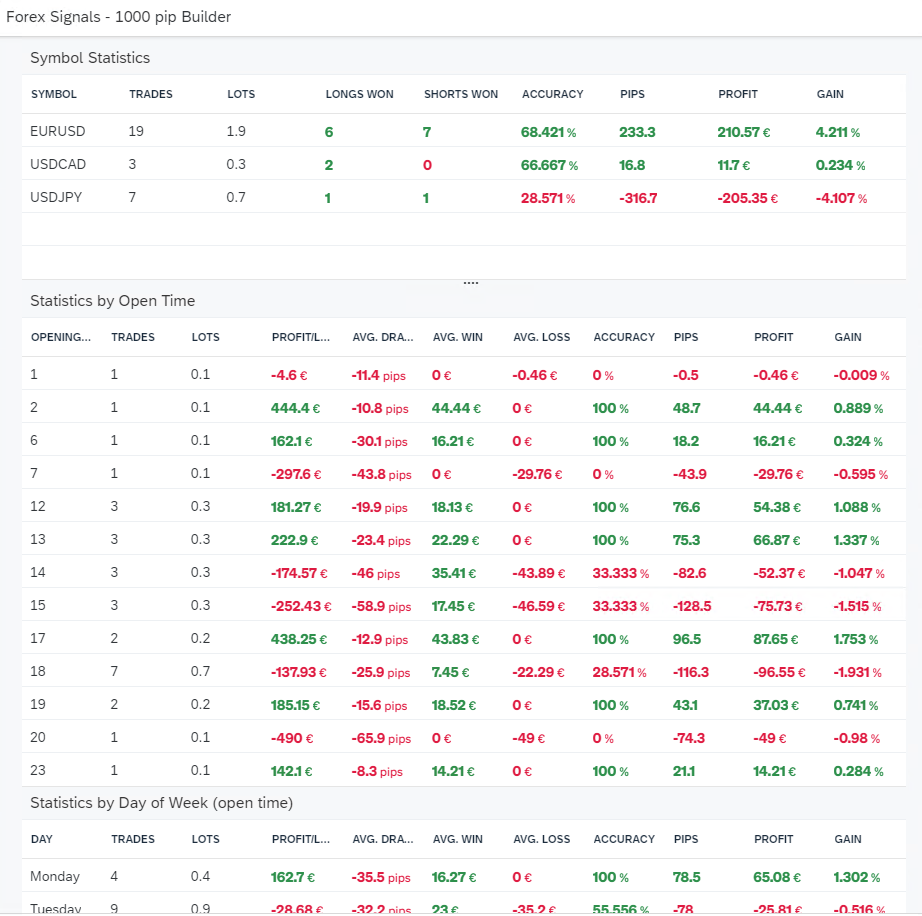This image is a screenshot featuring a detailed financial chart against a white background. At the very top left corner, in light gray font, the text reads "4x Signals - 1000 pip Builder." Directly beneath this, there is a very light grayish-blue border framing the chart.

The first section of the chart is titled "Symbol Statistics" in gray font. The headers for each column from left to right are: "Symbols," "Trades," "Lots," "Longs Won," "Shorts Won," "Accuracy," "Pips," "Profit," and "Gain." Under the "Symbols" header, the entries are "EUR/USD," "USD/CAD," and "USD/JPY."

Below this, another, more extensive chart is present, titled "Statistics by Open Time" on the left. The column headers in this chart, from left to right, are: "Opening Trades," "Lots," "Profits," "Average DRA," "Average Win," "Average Loss," "Accuracy," "Pips," "Profit," and "Gain." This section lists a long array of data, spanning 20 to 23 rows.

In both charts, numbers are color-coded: negative numbers appear in red, while positive numbers are in green, creating a mix of both positive and negative values.